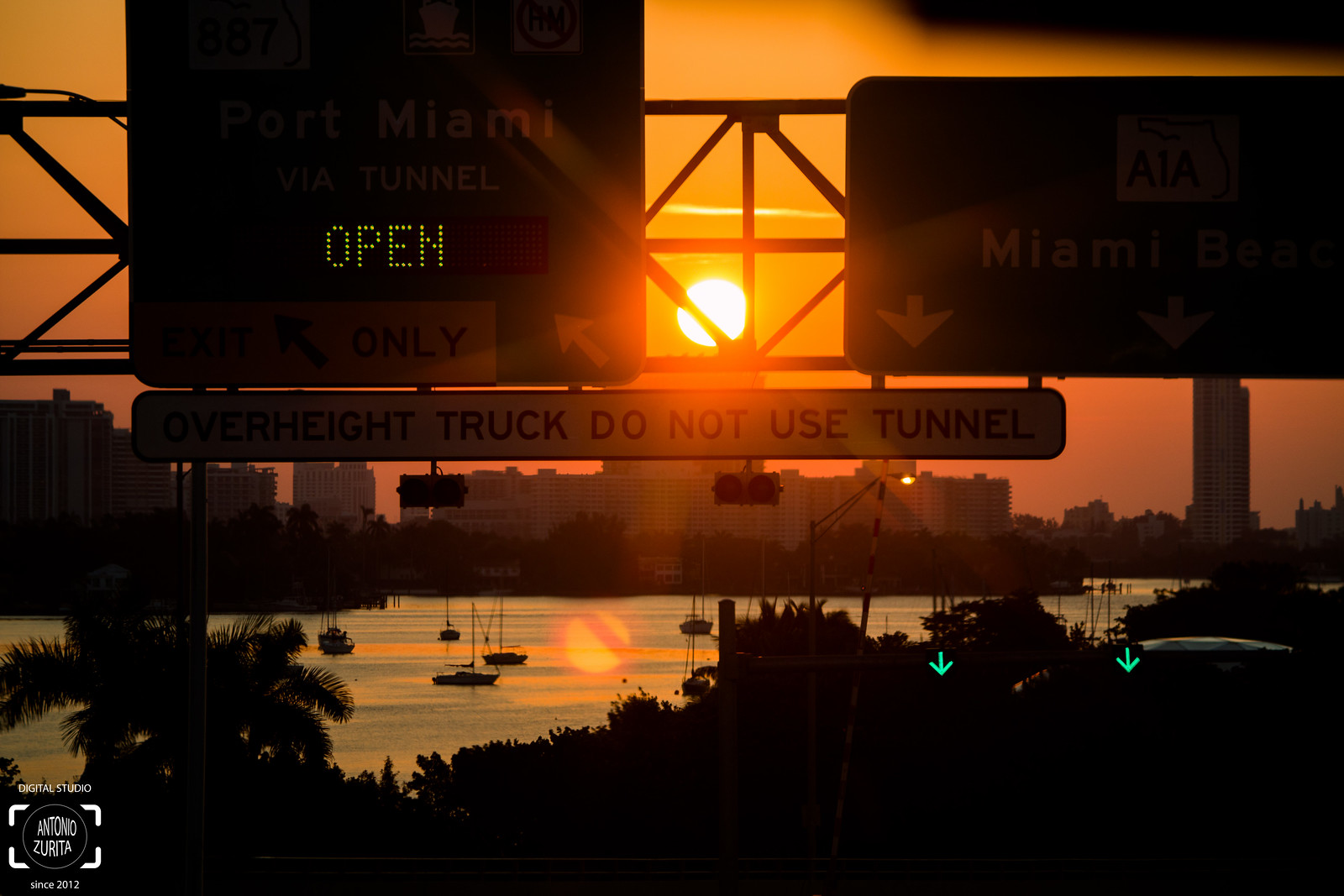The photograph captures a striking sunset over a lake, intersected by prominent highway signs in front of a distant city skyline. The sky is painted in hues of orange, transitioning to darker clouds as night approaches. Silhouettes of trees, buildings, and boats populate the serene water backdrop. The signs, though largely shadowed and indistinct, display some legible details: on the left, a green sign reads "Port Miami via Tunnel," accompanied by an illuminated LED screen with the word "Open" in green lights. Beneath that, a white sign warns, "Overheight Truck Do Not Use Tunnel." Adjacent to this, another green sign points towards "Miami Beach," featuring a small depiction of Florida with "A1A" marked on it, and white arrows directing the way. The metal support structure holding the signs cuts across the photo, adding a metallic element to the soft, natural beauty of the sunset-laden scene.